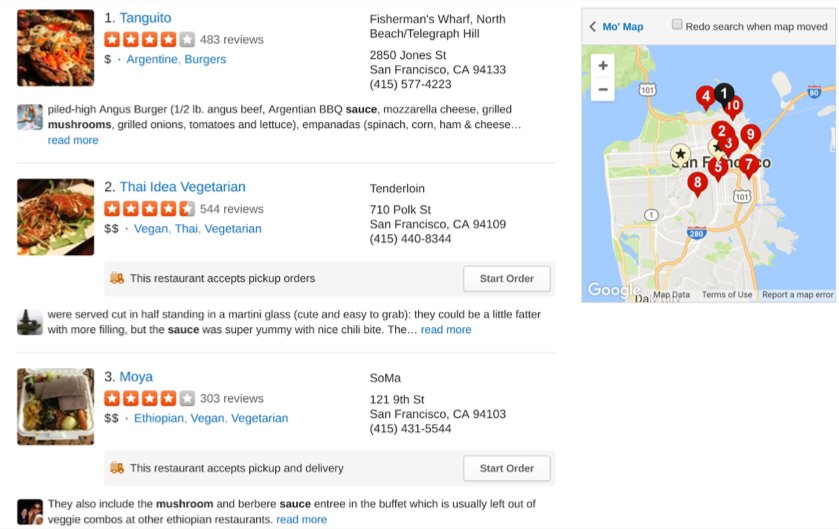This screen grab from Yelp.com presents a comprehensive guide to top-ranked restaurants in San Francisco. The layout features a white background on the left side, displaying three ranked restaurants, while the right side showcases a detailed map with red and black location markers indicating where these venues are located.

- **Tanguito**:
  - **Rating**: 4 stars out of 5.
  - **Price**: Single dollar sign ($), indicating it is on the less expensive side.
  - **Type**: Not specified, but implied to be well-rated.
  - **Address**: Listed.
  - **Review snippet**: Provided beneath the listing for quick insight.

- **Thai Idea Vegan**:
  - **Ranking**: Second.
  - **Rating**: 4.5 stars.
  - **Price**: Two dollar signs ($$), suggesting a moderately higher cost.
  - **Cuisine**: Vegan, Thai, Vegetarian.
  - **Address**: Included.
  - **Review snippet**: Available for additional context.

- **Moya**:
  - **Rating**: 4 stars out of 5.
  - **Price**: Two dollar signs ($$).
  - **Cuisine**: Ethiopian, Vegan, Vegetarian.
  - **Address**: Displayed.
  - **Review snippet**: Adds further information on what to expect.

The map to the right side complements the listings with red markers denoting the restaurants' locations and one black indicator for additional context. The map is colored light blue for water bodies and highlights that the area discussed is San Francisco.

Overall, the display is clean, symmetrical, and user-friendly, making it easy for viewers to discern key information about each restaurant at a glance.